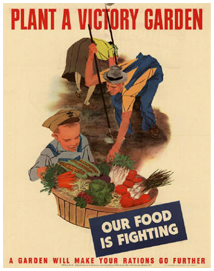This image depicts a World War I or World War II propaganda poster encouraging civilians to contribute to the war effort by planting victory gardens. At the top of the poster, bold red text reads "Plant a Victory Garden." Below, a blue rectangle contains white text that states, "Our Food is Fighting." Further down, small red letters say, "A garden will make your rations go further."

The central illustration features three figures diligently working in a garden. A woman, dressed in a brown skirt and a yellow top, is bent over pulling vegetables from the soil. Beside her, a man wearing blue overalls, a yellow shirt, and a gray hat performs similar tasks. Below them, a young boy or possibly a soldier in a blue outfit with a sailor-type hat proudly holds a large basket overflowing with tomatoes, corn, lettuce, and other vegetables. The background of the poster resembles aged, white paper, adding to the vintage feel of the image.